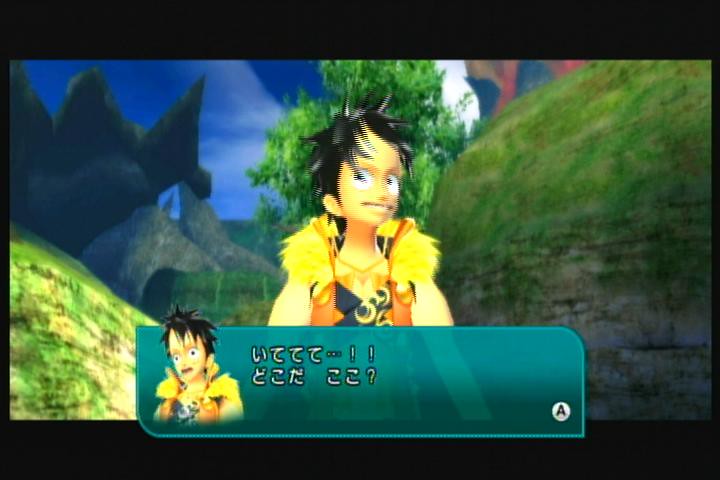A screenshot from a computer or video game depicts a vivid and engaging scene. Set against a pitch-black background, a teal text bubble occupies the bottom center of the image. The text within the bubble is rendered in a white font and written in a foreign language. The text bubble also contains an image of a female character featured in the screenshot. This character has spiky black hair and is adorned with a gold necklace. She wears a sleeveless top that boasts a striking combination of blue and red hues and is draped in a distinctive shawl made of yellow feather material. The setting is an outdoor grassy terrain, with dark gray mountains serving as a dramatic backdrop. To her left, a light green tree stands in stark contrast to the rugged landscape. Hills flank both sides of the scene, adding depth and context to her surroundings. The overall image is a captivating glimpse into the vibrant and dynamic world of the game.